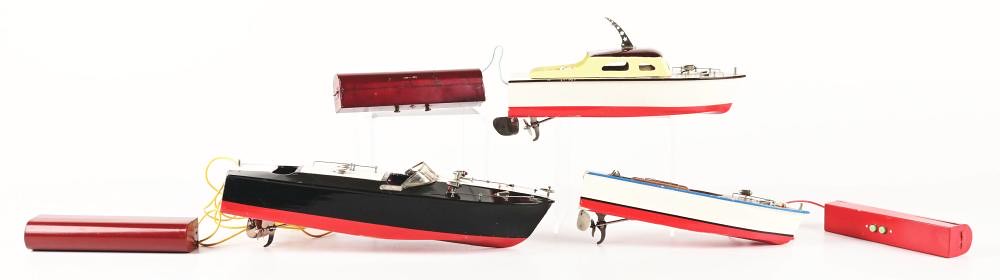This image depicts a set of three remote control boats arranged on a plain white background, each attached by a wire to distinct red battery packs that provide their power. The top boat features a sleek white hull with a black trim around the top and a red underside. It sports a distinctive yellow cabin with a black roof and a black shark fin adorned with white stars protruding from it, as well as a front gate. The middle boat, situated to the left, is entirely black with only the red bottom visible. It resembles a motorboat, equipped with a propeller and a simple window where the driver would sit, but lacks a cabin. Instead, it has a small area allocated for seating. The third boat, positioned on the bottom right, has a white hull with a blue rim around the top and a red base. This one also features a propeller fan on the bottom and defined seating areas. Each boat is intricately designed with attention to detail, from the coloration to the structural elements, clearly intended for controlled aquatic play or model display.